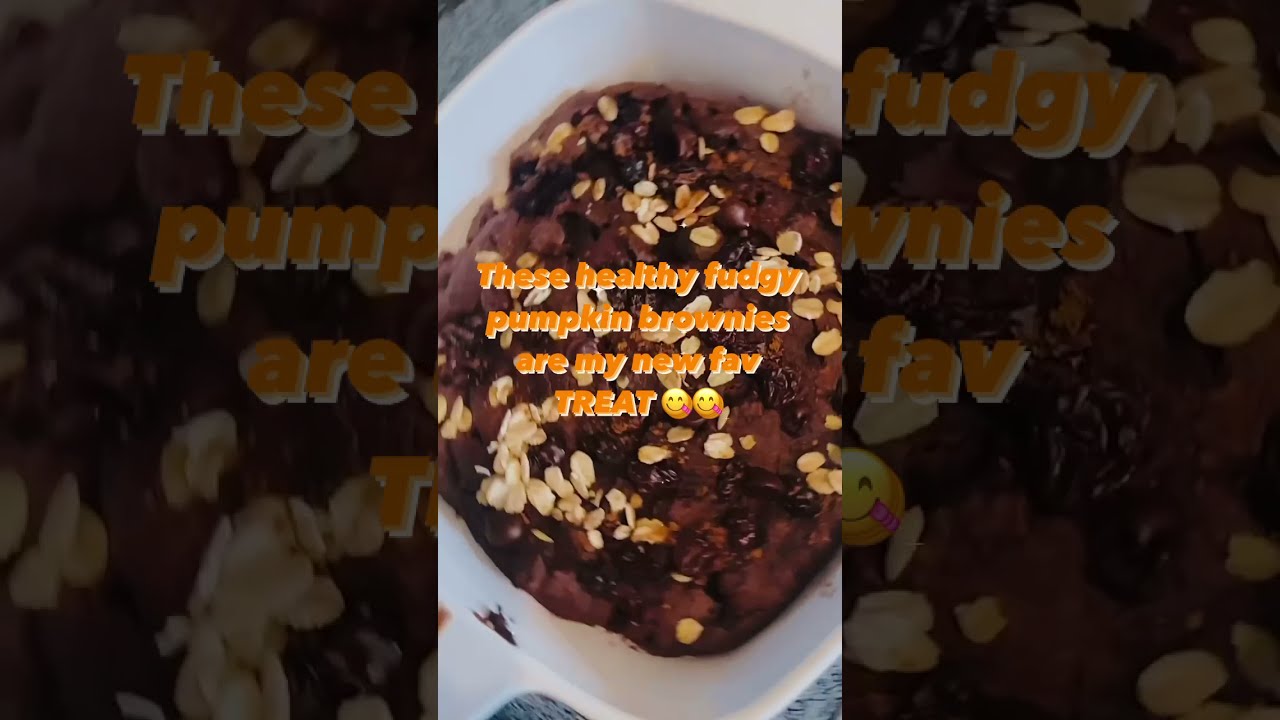The photo features a white dish filled with rich, brown fudge brownies, embedded with darker brown fudge pieces and sprinkled with white and yellow nuts, which may include pumpkin seeds. The middle of the image prominently displays orange and white text stating, "These healthy fudgy pumpkin brownies are my new fave treat," accompanied by two smiley face emojis with their tongues sticking out. The central panel is in sharp focus, highlighting the detailed texture of the brownies and their toppings. To the left and right, blurred, zoomed-in versions of the main image serve as a backdrop, providing an enhanced view of the fudge pieces, nuts, and emojis while filling the blank spaces on either side.